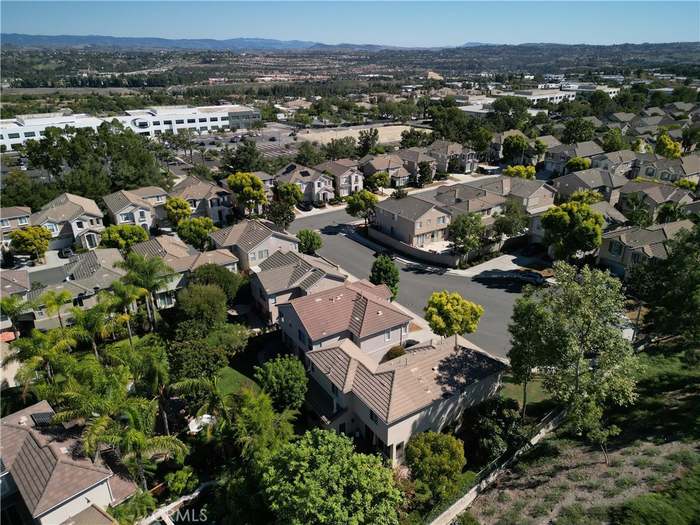This overhead drone photograph captures a sprawling residential neighborhood featuring large, uniformly designed two-story homes with beige and tan rooftops. The clean blacktop roads and light-colored sidewalks wind through this well-maintained community, characterized by lush, green yards and a variety of trees, including palm trees and native species. The bottom portion of the image is heavily lined with trees, while additional greenery is present in the backyards and around the houses, reinforcing the verdant atmosphere. To the horizon, there are hills and mountains that add a picturesque backdrop, underlining the subtropical yet somewhat dry setting, likely in California. Additionally, a tall, white building, possibly a warehouse, can be seen in the distant background. The image also features a watermark in the bottom left corner, reading 'CRMLS.' Indicating it as likely content related to real estate listings. The general ambiance suggests a modern, meticulously planned suburban area with a consistent architectural theme.